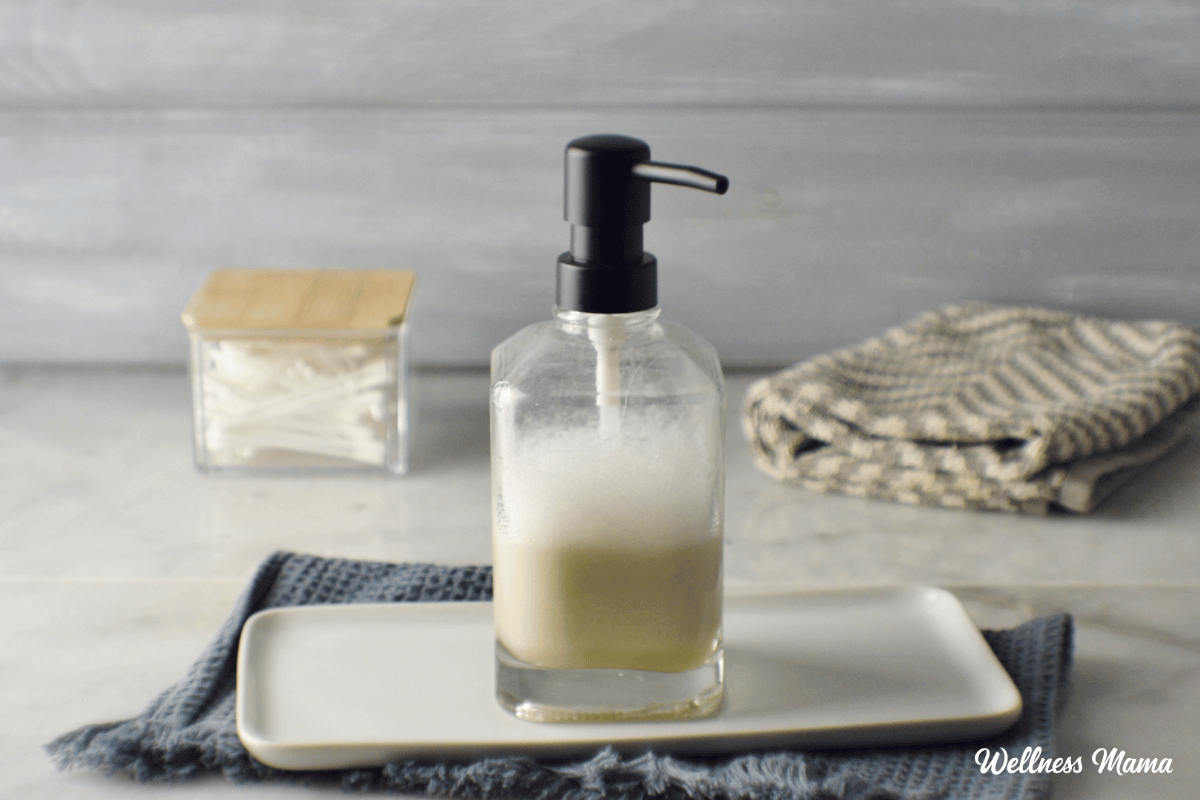The image depicts a detailed and organized bathroom counter. The counter itself is white, complemented by a grey background that gives a clean and minimalist appearance. Centrally placed is a glass lotion bottle with a black lid and a black pump, labeled "Wellness Mama" in white script on the bottom. The lotion inside is thick and creamy with a white internal dispenser. This bottle rests on a white rectangular plate, which in turn is on top of a neatly folded blue towel. Just behind the lotion, there is a folded yellow and grey washcloth. To the left, a glass container with a brown cover holds a collection of Q-tips, adding to the practical yet aesthetically pleasing arrangement. The overall setup, with its thoughtful placement of items like the folded grey and white-striped towel and minimalistic design, evokes a sense of a health and wellness setting, possibly curated for a lifestyle or beauty blog.